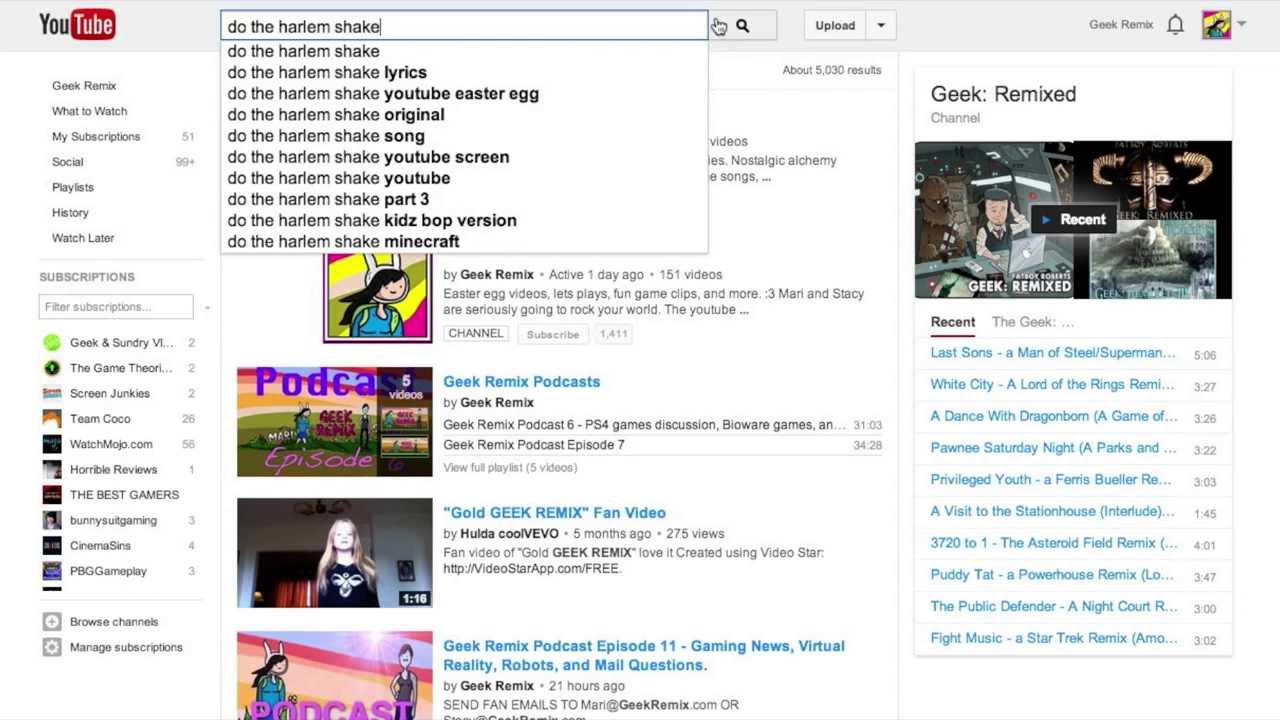In this nostalgic throwback to the YouTube platform of the 2000s, we observe the classic YouTube layout that many users fondly remember. On the left side, the iconic YouTube logo is prominently displayed, featuring a bold, black "U" in Impact font followed by "Tube" in white letters, encased within a red rectangular background. This emblem stands out against the white backdrop of the site, drawing the viewer's eye.

Moving to the right, we notice the search bar containing the text query, "Do the Harlem Shake," written in Arial Black font. Adjacent to the search bar, the cursor is placed at the far right, bringing attention to the dropdown box filled with various search suggestions. The suggestions include options like "Do the Harlem Shake," "Do the Harlem Shake Lyrics" (with "Lyrics" highlighted in bold), "Do the Harlem Shake YouTube Easter Egg" (with "YouTube Easter Egg" in bold), "Do the Harlem Shake Original" (with "Original" in bold), and several other variations, each with specific keywords emboldened for emphasis.

Next to the search bar, we see an illustrated Disney hand, recognizable by its glove, with the thumb and index finger extended as if to click. Following this, there's a black magnifying glass icon representing the search function. Beside these elements, a small gray rectangle with the word "Upload" in dark gray text indicates the button for uploading videos. To its right, a gray square with a downward-pointing arrow suggests a dropdown menu for additional options.

Further right, small gray Arial font text reads "Geek Remix," denoting the user's channel or account name. A bell icon outline signifies the notification area, alerting users to recent updates or interactions. Finally, a user icon with a red background is seen, indicative of the user profile section.

Beneath the YouTube logo on the left side, the white background continues into a menu listing several functional options such as "Geek Remix," "What to Watch," "My Subscriptions," "Social," "Playlist," "History," and "Watch Later," each option leading users to different sections of the platform for easy navigation.

This detailed depiction captures the essence of YouTube's interface during a memorable era, evoking a sense of digital nostalgia.